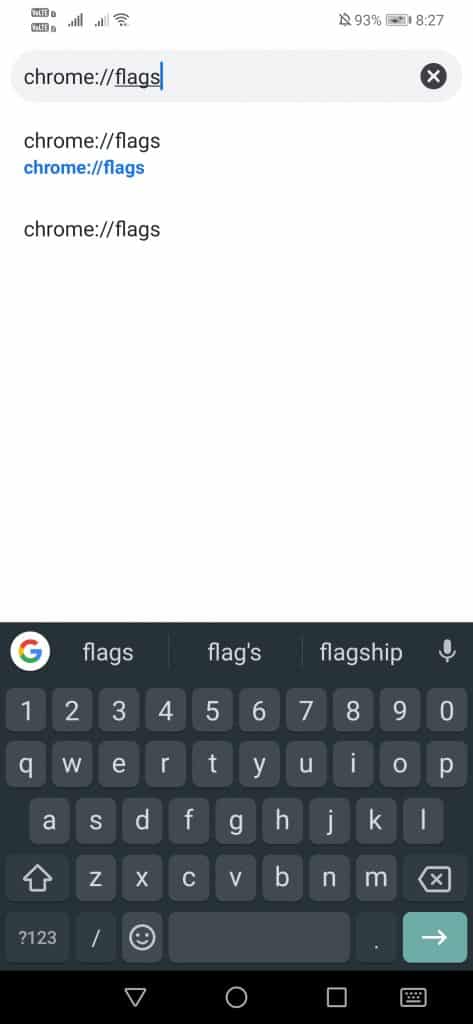The screenshot depicts an Android smartphone screen captured at 8:27 (specific time format unmentioned). The battery icon indicates a 93% charge, and the phone is set to silent mode. At the top left, multiple cell signal icons are visible, suggesting the phone operates on two networks, possibly utilizing dual SIM cards—one for Verizon and another for T-Mobile, both connected via LTE. One signal shows full strength with five bars, while the other has three bars; a single Wi-Fi signal icon is also present.

Centrally, the browser's address bar displays "chrome://flags" repeated three times, with the third instance highlighted in blue, likely signifying a user-specific action or search. At the screen's bottom, the virtual keyboard is visible, featuring both alphabetical and numeric keys. Navigation icons—a downward triangle, a circle, and a square—are also shown alongside a keyboard icon. The keyboard is in lowercase mode, and above it, Google’s logo appears with predictive text suggestions: "flags," "flags'," and "flagship." This setup suggests the user is exploring or customizing Chrome browser settings on their smartphone.